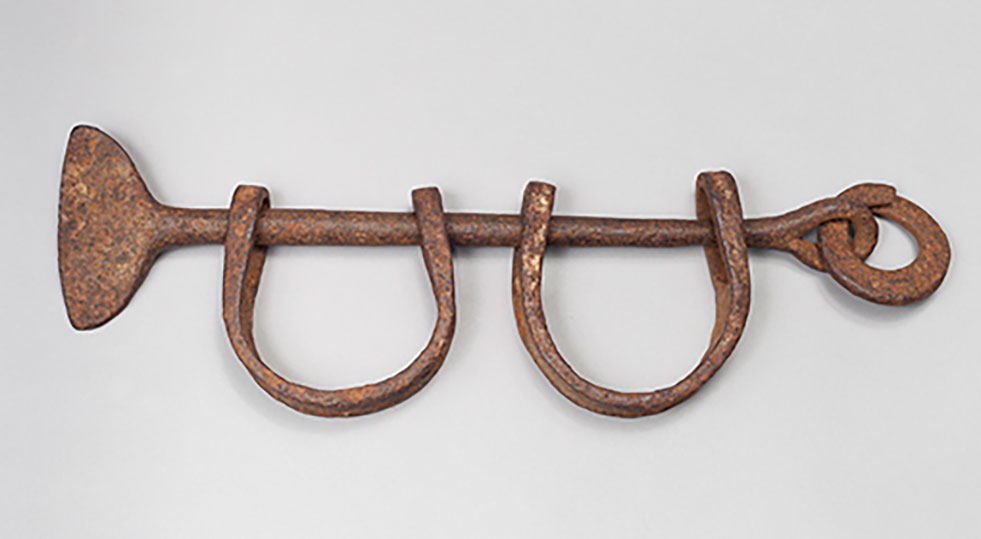The image depicts an antique, rusted metal rod, horizontally positioned against a gray or white background. The rod features distinctive elements: at the left end, there is a paddle-like or squared-off spoon shape, while the right end concludes in a rounded point with a circular ring attached, forming a loop. Suspended along the middle of the rod are two horseshoe-shaped metal pieces, also showing signs of rust. The horseshoe-like objects seem to be attached by sliding over one end of the rod, lying next to each other. This arrangement suggests a decorative or possibly historical tool, with the entire assembly hinting at a utilitarian purpose from a bygone era. The lighting in the image creates subtle shadows, especially on the left side, adding to the aged and worn appearance of the metal.